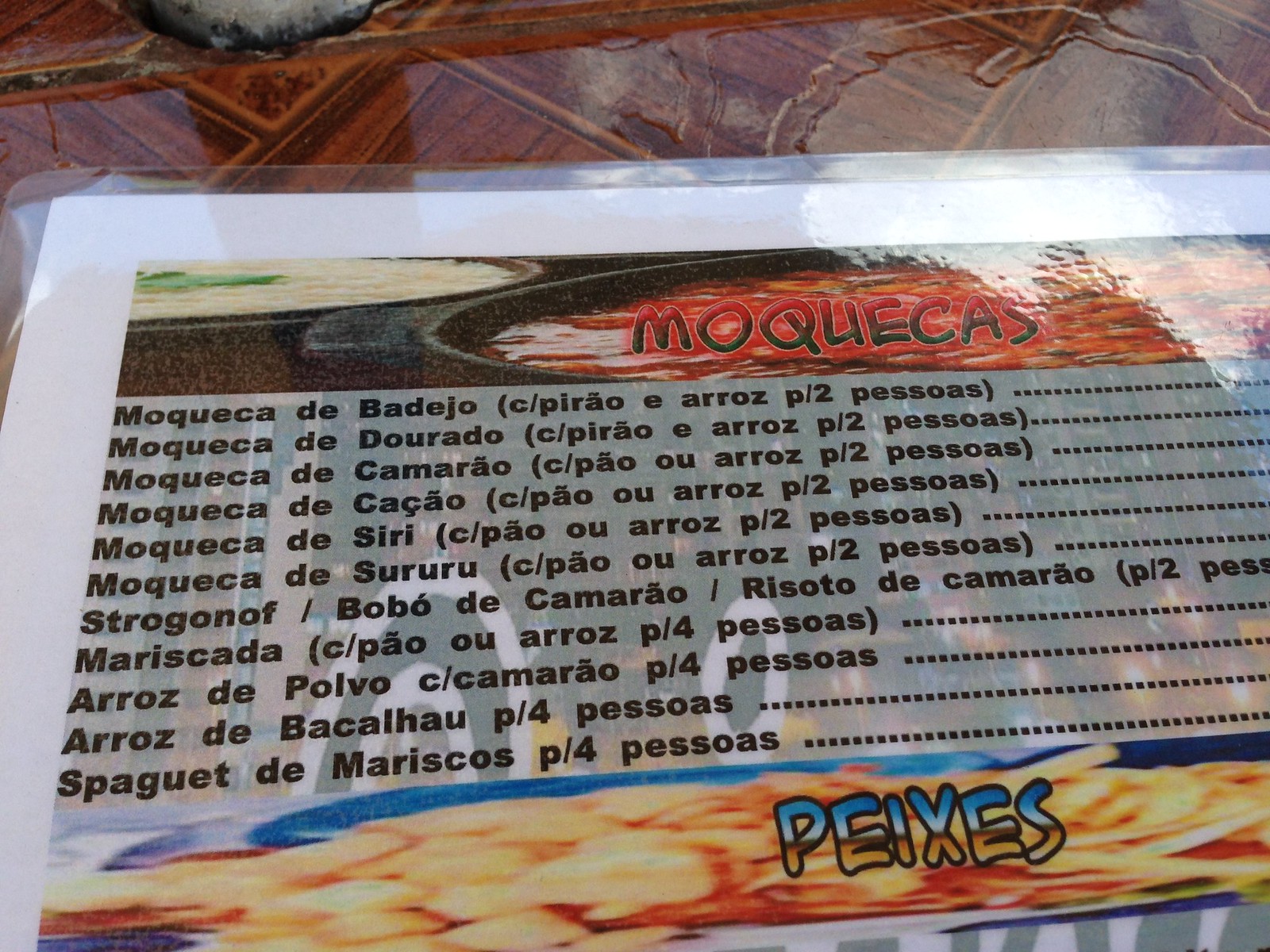The photograph depicts a laminated, glossy menu placed on a richly hued wooden table. The menu, primarily written in what appears to be Spanish, showcases various dishes with detailed descriptions but no visible prices. Under the heading "MOQUECA," followed by choices like "Moqueca de Badejo," about ten items are listed. Additionally, the menu features a second heading, "PEIXES," indicating various types of fish dishes. Scattered across the menu are colorful illustrations of bowls containing salsas or chili, and another bowl full of rice, enhancing the visual appeal. The overall setting is warm and inviting, emphasizing the traditional and vibrant culinary offerings.